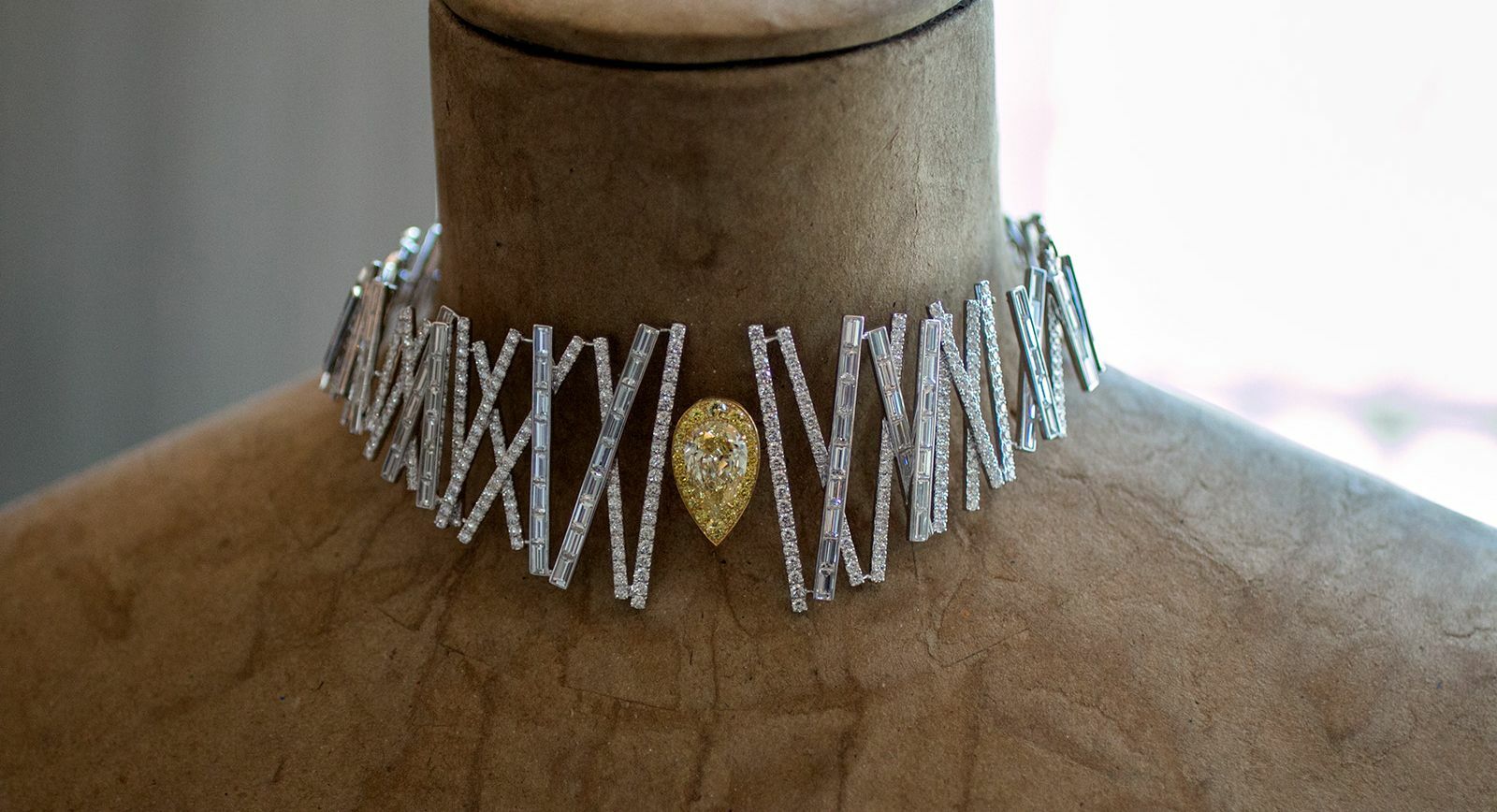This professional photograph, likely used for advertising, showcases an intricate, bold choker necklace displayed on a headless mannequin, captured from an up-close, horizontal perspective. The mannequin, only showing the neck and shoulders, features a textured brown velvet or tan suede finish, providing a rich backdrop for the jewelry. The centerpiece of the necklace is a gold teardrop-shaped gem, possibly replicating a yellow diamond, surrounded by small round diamonds. Extending from this central piece are strips of diamonds arranged in a series of crisscrossing 'X' patterns that progressively diminish in size toward the edges. The X's consist of both round and square baguette-style diamonds, creating a striking and garish visual impact.